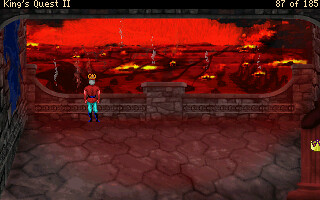The image depicts a scene from the classic DOS computer game, King's Quest II. The upper left-hand corner displays "King's Quest II" in white text, while the upper right-hand corner shows the score "87 of 185". The setting appears to be inside a castle or dungeon, characterized by gray and purple shaded, scaly-type ground. A small character with a golden crown, red jacket, light blue pants, and dark blue boots stands in the foreground, facing away from the viewer. The background reveals a dramatic volcanic landscape with erupting volcanoes under a blood-red sky. A series of lava holes with yellow and orange spots enhance the fiery ambiance, and a solitary pillar crowns the right side of the scene.